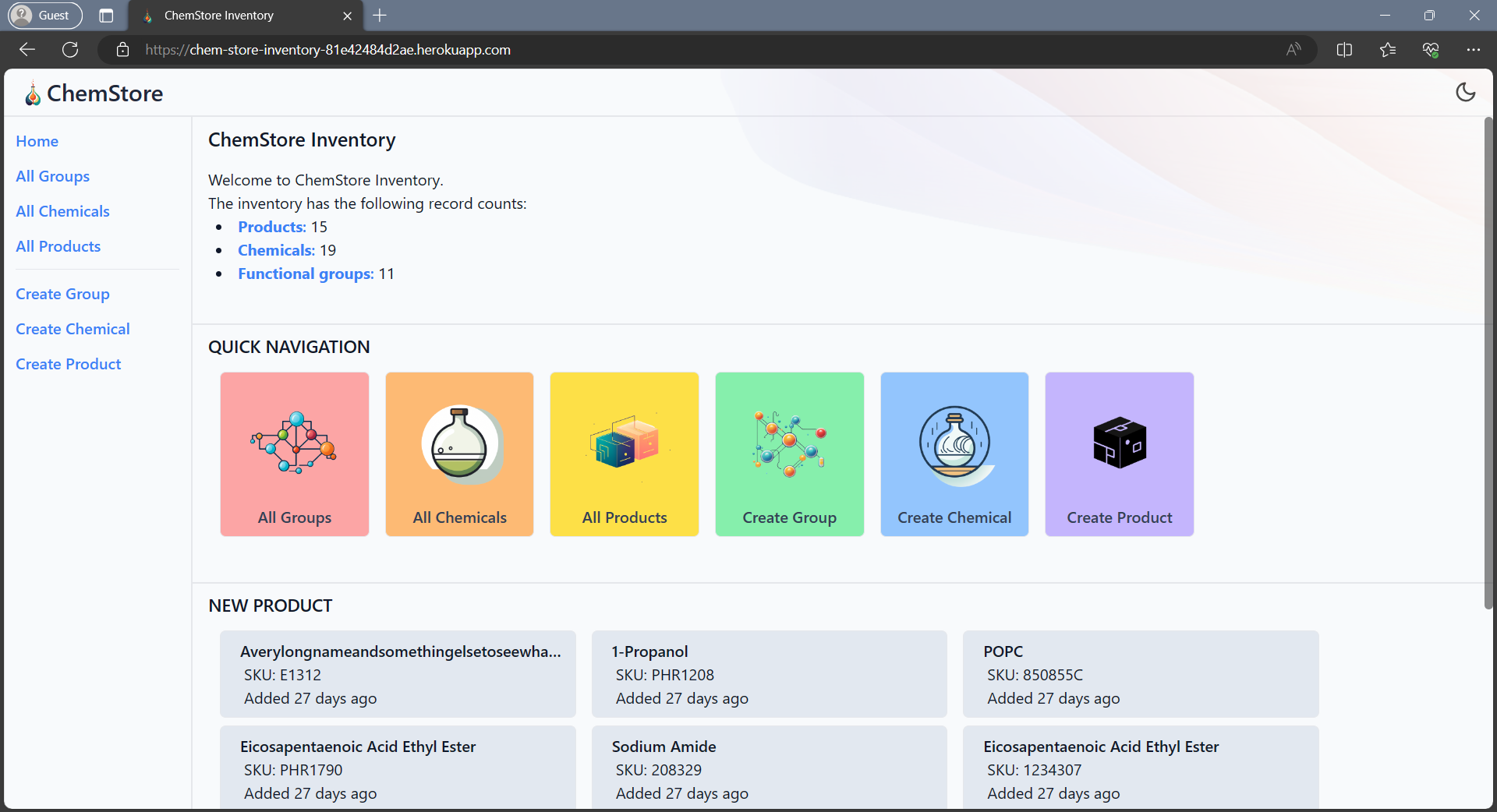This image is a screenshot of a desktop web browser, most likely Google Chrome, running on a Windows or Linux operating system, based on the presence of the typical window control icons (X, minimize, and maximize) in the top right corner. The user is browsing in Guest mode, as indicated by the interface. The URL in the address bar is "https://chem-store-inventory-81e42484d2ae.herokuapp.com", which takes you to a website named ChemStore Inventory.

The website welcomes visitors with the headline "ChemStore Inventory" and an introductory message stating, "Welcome to ChemStore Inventory." It presents a summary of inventory records displaying the quantities: Products (15), Chemicals (19), and Functional Groups (11).

On the left side of the interface, there is a navigation menu with various options:
- **Home**
- **All Groups**
- **All Chemicals**
- **All Products**
- **Create Group**
- **Create Chemical**
- **Create Product**

Below the navigation menu, there's a "Quick Navigation" section featuring different icons with illustrative images:
- **All Groups**: Red background with a multicolored molecular structure.
- **All Chemicals**: Orange background with an old potion vial containing green fluid.
- **All Products**: Yellow background with green and orange square boxes.
- **Create Group**: Light green background with another molecular symbol.
- **Create Chemical**: Pale blue background with a potion bottle featuring wind and raindrop elements.
- **Create Product**: Pale purple background with a black box.

The main content area shows a list of recently added products, each accompanied by an SKU and information on when they were added. The products listed include:

1. **Avery long name and something else to see what...**
   - SKU: E1312
   - Added: 27 days ago

2. **1-Propanol**
   - SKU: PHR1208
   - Added: 27 days ago

3. **POPC**
   - SKU: 850855C
   - Added: 27 days ago

4. **Eicosapentaenoic Acid Ethyl Ester**
   - SKU: PHR1790
   - Added: 27 days ago

5. **Sodium Amide**
   - SKU: 208329
   - Added: 27 days ago

6. **Eicosapentaenoic Acid Ethyl Ester** (listed again with a different SKU)
   - SKU: 1234307
   - Added: 27 days ago

The website ChemStore appears to sell various chemicals and related products, likely catering to scientific and industrial needs.